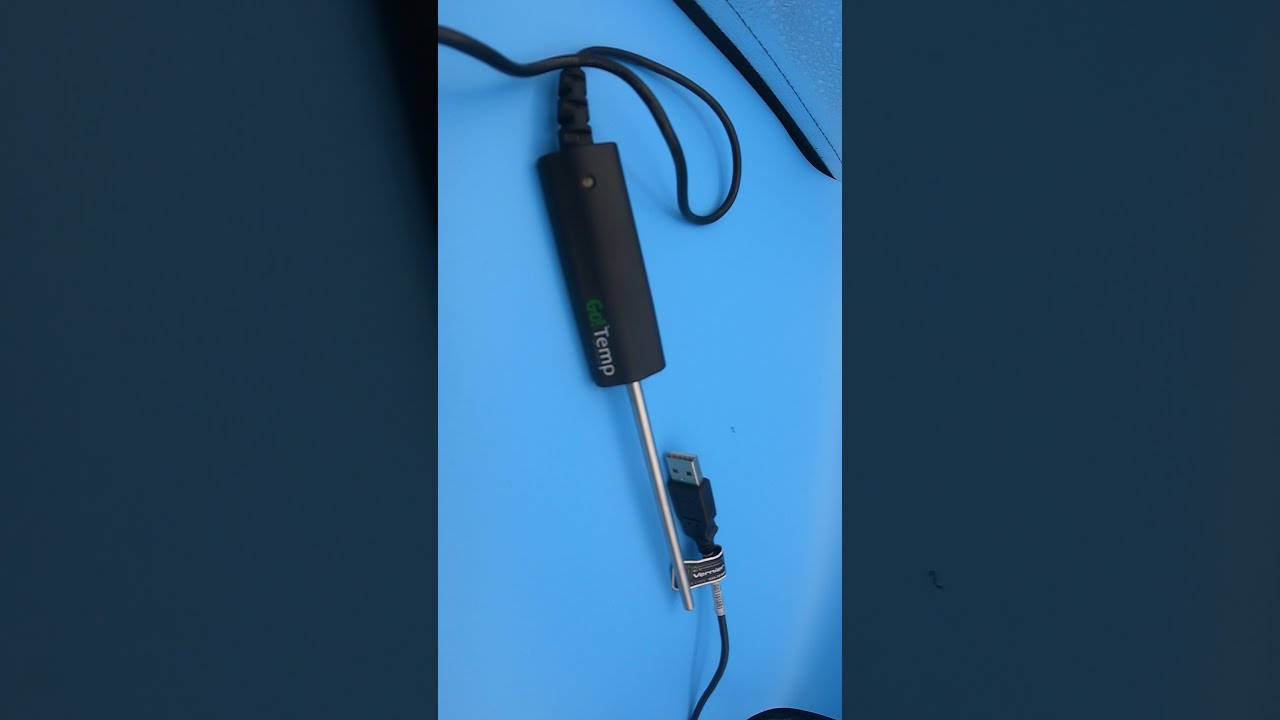The image depicts an electronic temperature probe device positioned centrally on a dark blue surface with a lighter blue strip running horizontally across the middle. The device features a large round black handle ending in a pointed silver metallic rod, attached to a black rectangular plastic component labeled "Go Temp" in green and white text. Connected to the handle is a wire extending towards the top left corner of the device. Below the device, a USB cable with a black tag and white lining runs towards the bottom of the image. Additionally, two large dark blue rectangles can be seen on either side of the image, framing the setup. An extra black wire runs along one corner, adding to the intricate layout of the scene.